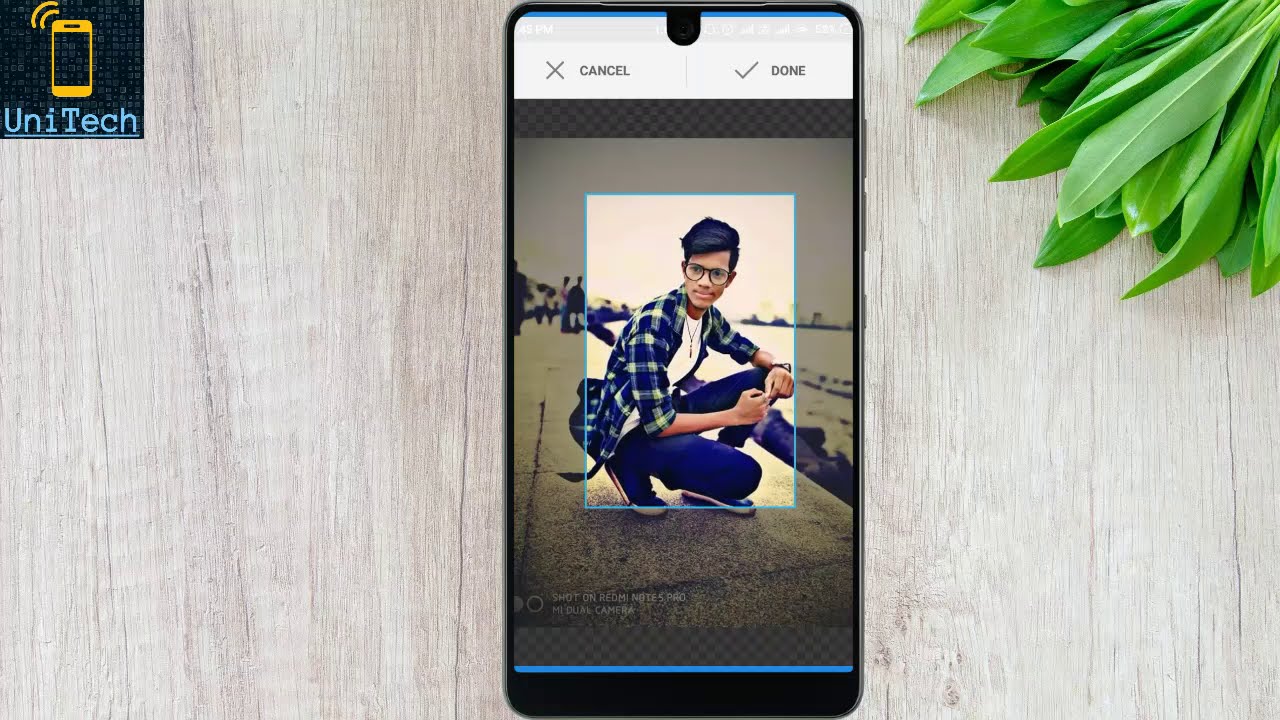In the center of the image, there is a cell phone lying on a white wooden table. On the screen of the cell phone, the picture portrays a young man, possibly a teenager or in his early twenties, squatting on a sidewalk near what appears to be a body of water. He has black hair and is wearing round, black glasses, a white T-shirt, blue and white flannel, purple-blue jeans, and running shoes. The man is looking to the left, with a washed-out white sky and distant land in the background.

At the top of the cell phone screen, there are two options: an "X" labeled "cancel" on the left and a checkmark labeled "done" on the right, both against a white strip. The border of the cell phone screen features a checkerboard pattern of black and lighter gray squares, with a blue stripe along the bottom. In the upper left corner of the cell phone screen, a yellowish outline of a cell phone is displayed with the text "Unitech" written in blue beneath it. In the upper right section of the image, some dark green laurel-like leaves are visible, suggesting the presence of a plant.